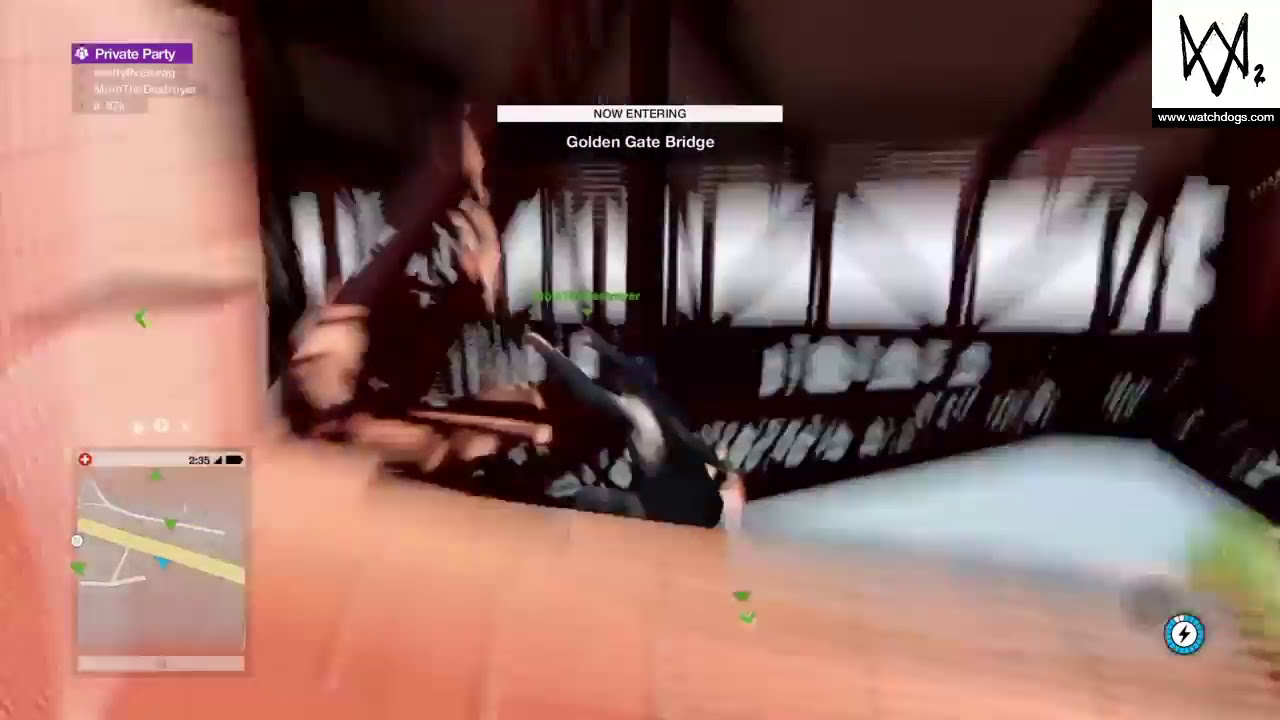This screenshot from the video game "Watch Dogs" features a blurry image capturing the action-packed scene under the Golden Gate Bridge. A character, possibly engaging in some form of communication with their left hand up to their face, is visible, holding an indiscernible weapon in their right hand. The game's interface overlays the screen, detailing context and in-game information. At the top left corner, there is a purple banner reading "Private Party," while the bottom left corner shows a small inset map, indicating the player’s position with a battery meter and a time display of 2 minutes and 35. Central to the image, a white bar with black text states "now entering," followed by a black bar with white text that reads "Golden Gate Bridge," confirming the iconic location. The top right corner features a logo and the URL www.watchdogs.com. The scene, though extremely blurry, hints at a tense moment under the bridge, likely involving a high-stakes infiltration or action sequence.